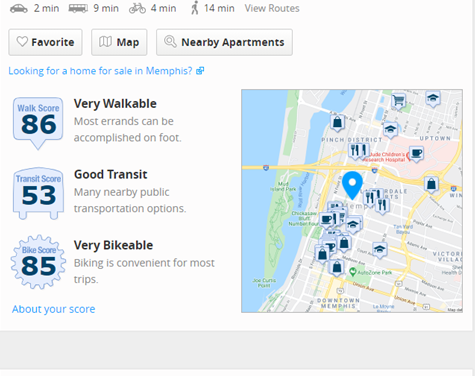This slightly rectangular, horizontally-oriented screenshot is from a travel or destination information app. At the top of the image, a bar displays various forms of travel options with their respective times: driving (2 minutes), public bus or transportation (9 minutes), biking (4 minutes), and walking (14 minutes). There's also an option to view routes. Below this, three side-by-side buttons are labeled 'Favorite,’ ‘Map,’ and ‘Nearby Apartments.’

Presented further down, a text box inquires, "Looking for a home for sale in Memphis?" Directly underneath, it states the area is "very walkable," indicating that most errands can be accomplished on foot, with an impressive walk score of 86. The transit score is 53, suggesting good transit options with many nearby public transportation choices. The bike score is 85, pointing out that the area is very bikeable and biking is convenient for most trips.

On the right side of the frame, a map displays various location icons for restaurants, shopping centers, schools, etc. A blue, upside-down teardrop pinpoints a specific location, although the map doesn't clearly indicate the exact area.